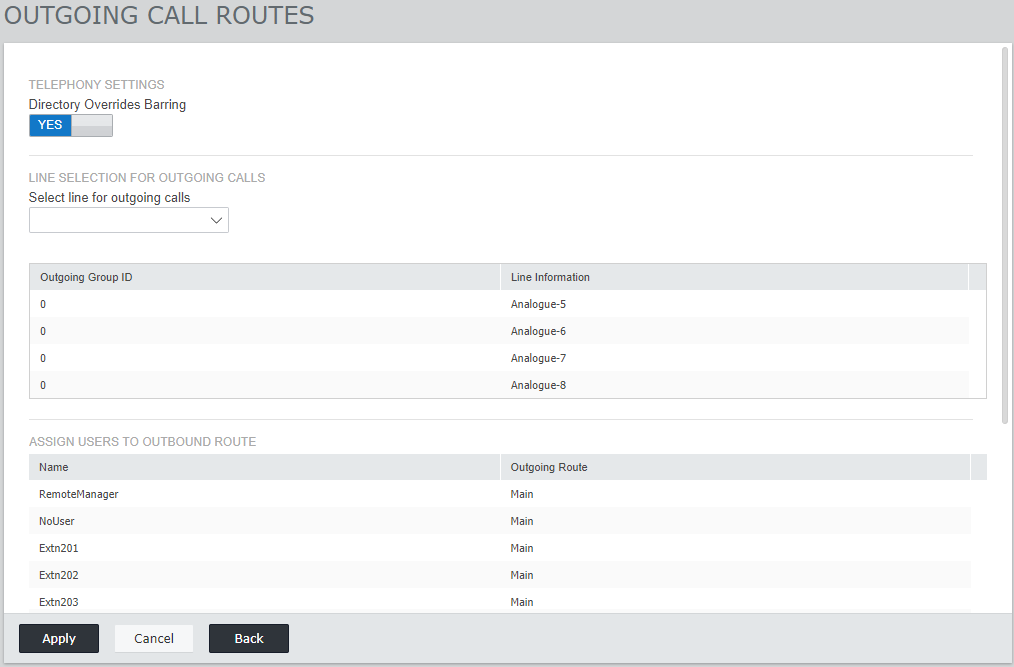The image is a screenshot of a settings page, titled "OUTGOING CALL ROUTES" in black, capital letters located at the top left corner of the page, close to both the top and left edges. 

Below this, there is a white section with some padding. At the top of this white area, positioned with notable spacing from the borders, it reads "Telephony Settings" in gray font. 

Underneath this, the text "Directory Overrides Bearing" appears in black font, followed by a status indicator that reads "YES" inside a blue box with white font.

The next section below is labeled "Line Selection for Outgoing Calls." Within this section, it states "Select Line for Outgoing Calls" next to an empty drop-down selection box. Further down, another field is labeled "Outgoing Group ID."

At the bottom of the page, three buttons are arranged horizontally: "Apply," "Cancel," and "Back."